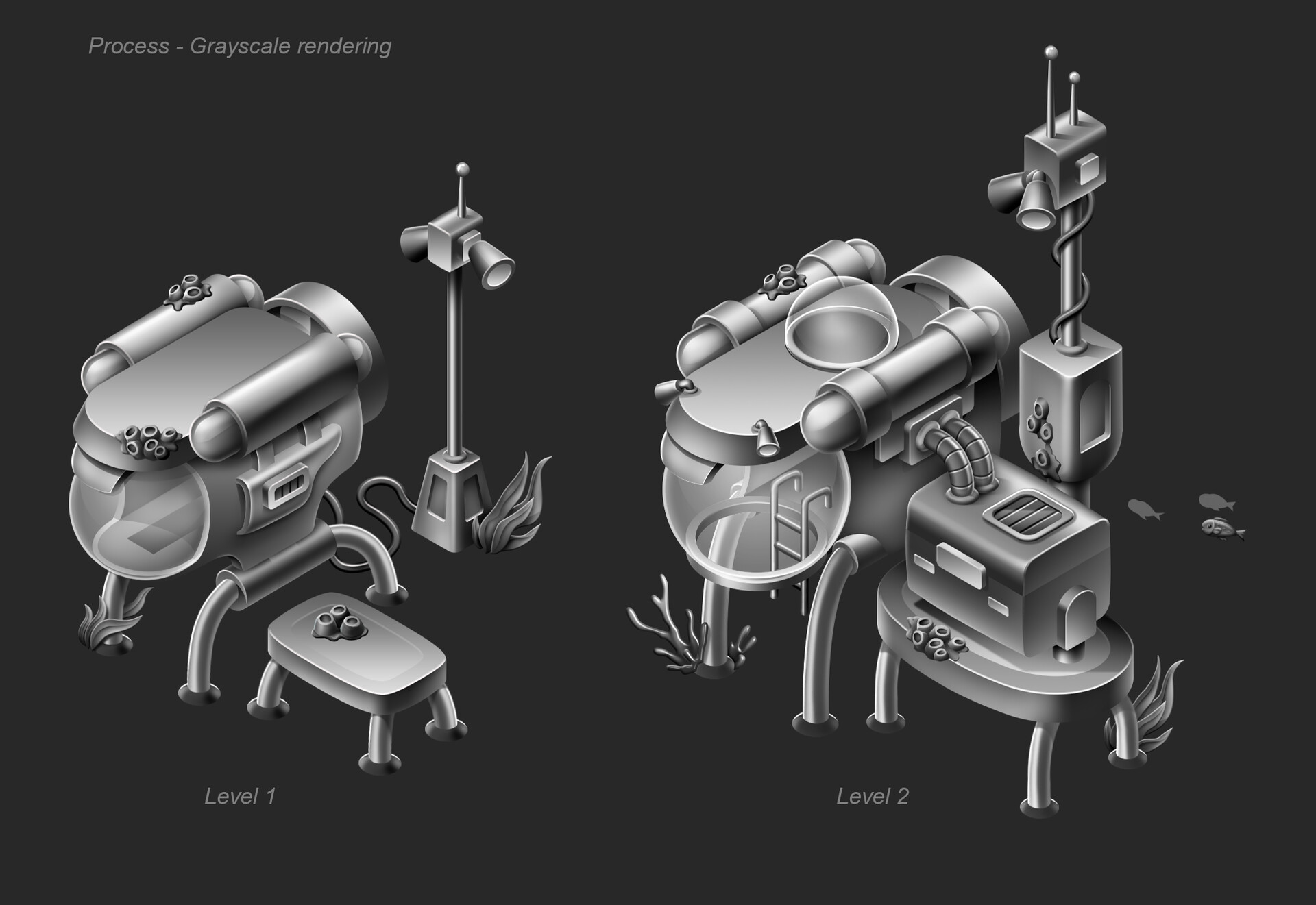The image is a detailed grayscale rendering or blueprint of two levels of a nautical structure set against a pitch-black background. At the top left, it features the small gray text "Process-GrayscaleRendering." The rendering is split into two sections labeled as "Level 1" on the left and "Level 2" on the right. 

Both sections depict a submarine-shaped craft resting on four downward-curving legs. In "Level 1," the structure includes a basic tank supported by legs, with a small table in front of it featuring similar legs, and a cord that connects to a light post. "Level 2" showcases a more detailed and complex design, with the same tank now featuring a hole at the bottom connected to a submarine-like piece with a ladder extending inside. The table houses a box with tubes running to the main tank, and a bubble dome at the top allows for additional observation. Additionally, the light post on the right is more elaborate, with a larger box, stronger cable, and attached lights. The background of "Level 2" also includes a small school of fish, hinting at a marine environment.